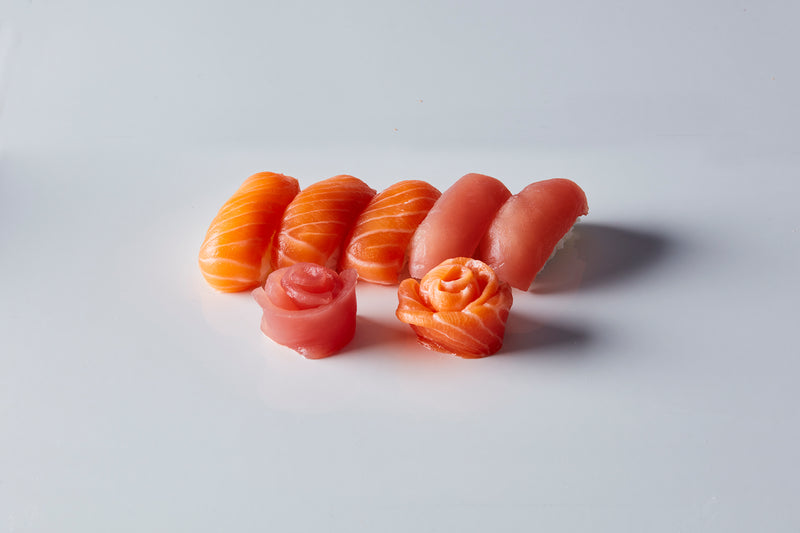The image depicts a culinary presentation against a subtly varying gray background, highlighting the light play and casting soft shadows. Centrally positioned are seven pieces of sushi, meticulously arranged. The back row features a horizontal alignment of five pieces: three are orange with distinct white stripes, typical of salmon, while the remaining two are a lighter pink, suggesting tuna. In the front, two pieces curl gracefully into rose shapes; the left rose is pink, resembling tuna, and the right rose is orange with white stripes, characteristic of salmon. A glimpse of rice is visible beneath the leftmost piece in the back row, enhancing the sushi's authenticity. The precise arrangement and the interplay of colors and textures emphasize the artistry involved in sushi preparation.